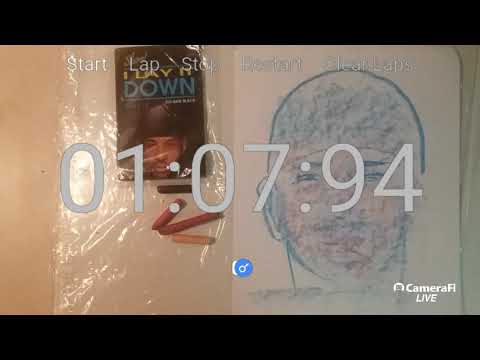The image appears to be a still shot, likely from a screenshot, of an application called Camerify Live, indicated by the logo "CAMERAIFY LIVE" in white font on the bottom right corner. The image has long, horizontal black bars along the top and bottom, giving it a letterboxed appearance. Overlaid on the black bar at the top, there are white font labels reading "start," "lap," "stop," "restart," and "Leak Labs." In the middle of the image, there is a time stamp "01:07:94" in large white letters, which could be a timer.

The main content of the image features two items side by side on a table. On the left, there is a book or novel wrapped in plastic titled "I Lay It Down," featuring the face of a black man on its cover. To the right of the book, there is a sketch of the same man on an 8.5 by 11 sheet of white paper, drawn in blue crayon or pencil. Also visible is a box, possibly related to the book, and a plastic bag that appears to contain either cigarette butts or blunts, suggesting it might be for ethnic hair care due to its proximity to the book themed around ethnic identity.